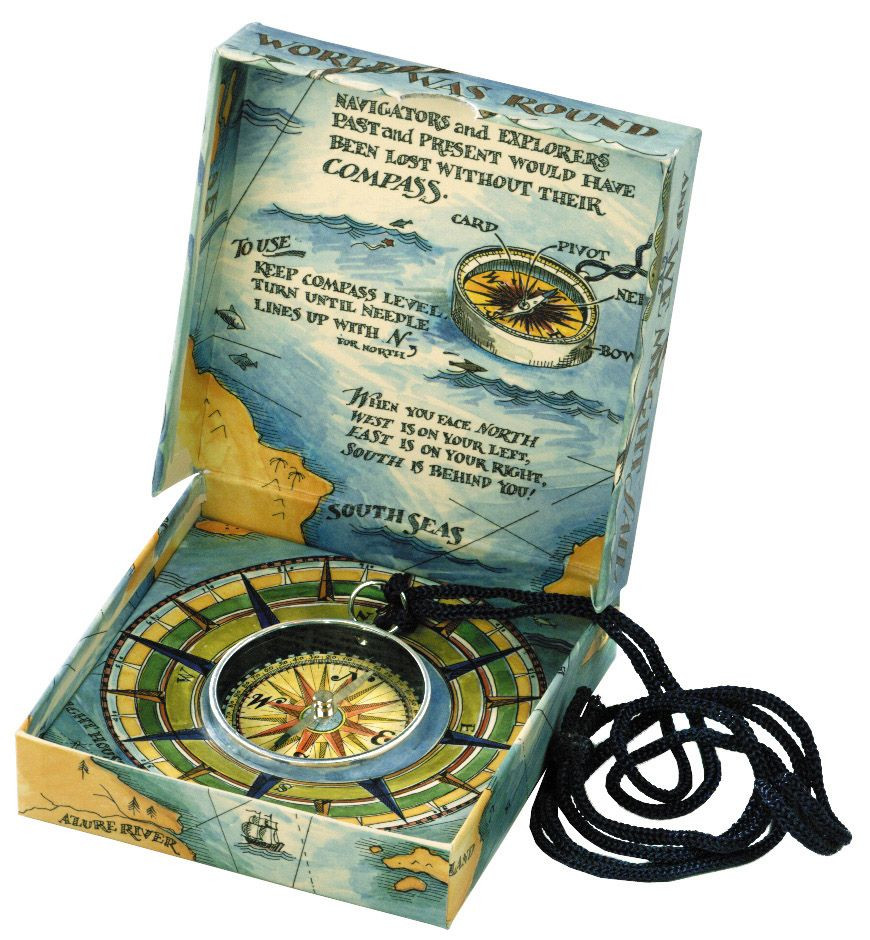This close-up image showcases a beautifully decorated wooden box designed to hold a compass. The box is painted with vibrant depictions of seas, landmasses, waves, fish, and sailing ships, creating a charming and detailed maritime theme. In the center of the open box rests a compass on a coiled black rope, designed for easy carrying or wearing around the neck. The inner lid of the box features a nostalgic inscription: "Navigators and explorers past and present would have been lost without their compass," along with practical instructions for using the compass: "Keep compass level, turn until needle lines up with N for north. When you face north, west is on your left, east is on your right, south is behind you." Additionally, the compass and some of its points are artistically depicted on the box, further emphasizing its navigational purpose. The top of the box bears the words "World was round," encapsulating the spirit of exploration. The predominant colors are blue, tan, black, silver, and red, enhancing the box’s aesthetic appeal.